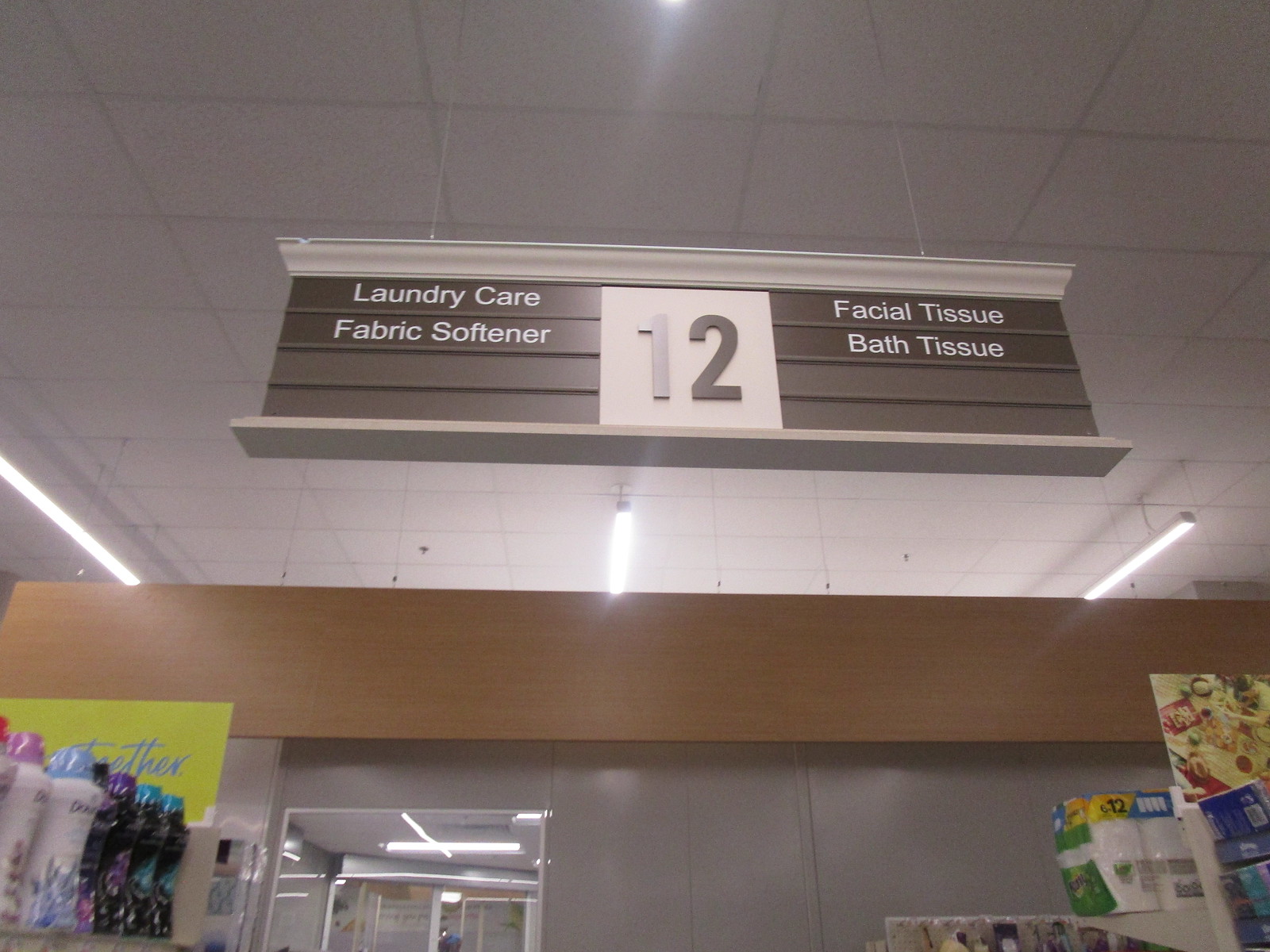The image captures a view from below of an aisle sign hanging from the ceiling in a grocery store. The sign is a large rectangular panel with a prominent white square in the center, displaying the number "12" in bold brown numerals. On the left side of the sign, two horizontal slats hold labels, with "Laundry Care" at the top and "Fabric Softener" underneath. Similarly, the right side of the sign features four horizontal slats designed to hold labels, with "Facial Tissue" at the top and "Bath Tissue" at the bottom. A white border frames the top and bottom edges of the sign.

The sign is suspended from the white-tiled ceiling by two small silver chains—one on the left and one on the right. In the background, the ceiling is fitted with fluorescent light fixtures, visible towards the left, center, and right sides of the image. 

In the foreground, the bottom left corner shows a shelf stocked with various colored bottles of Downy Unstoppables. On the right side of the image, the back of a 12-pack of Bounty Paper Towels is visible. Directly in the center of the photo, behind the aisle sign, there is a structure with brown siding on the upper half and gray siding on the lower half, with a small doorway that likely leads to an office or restroom area.